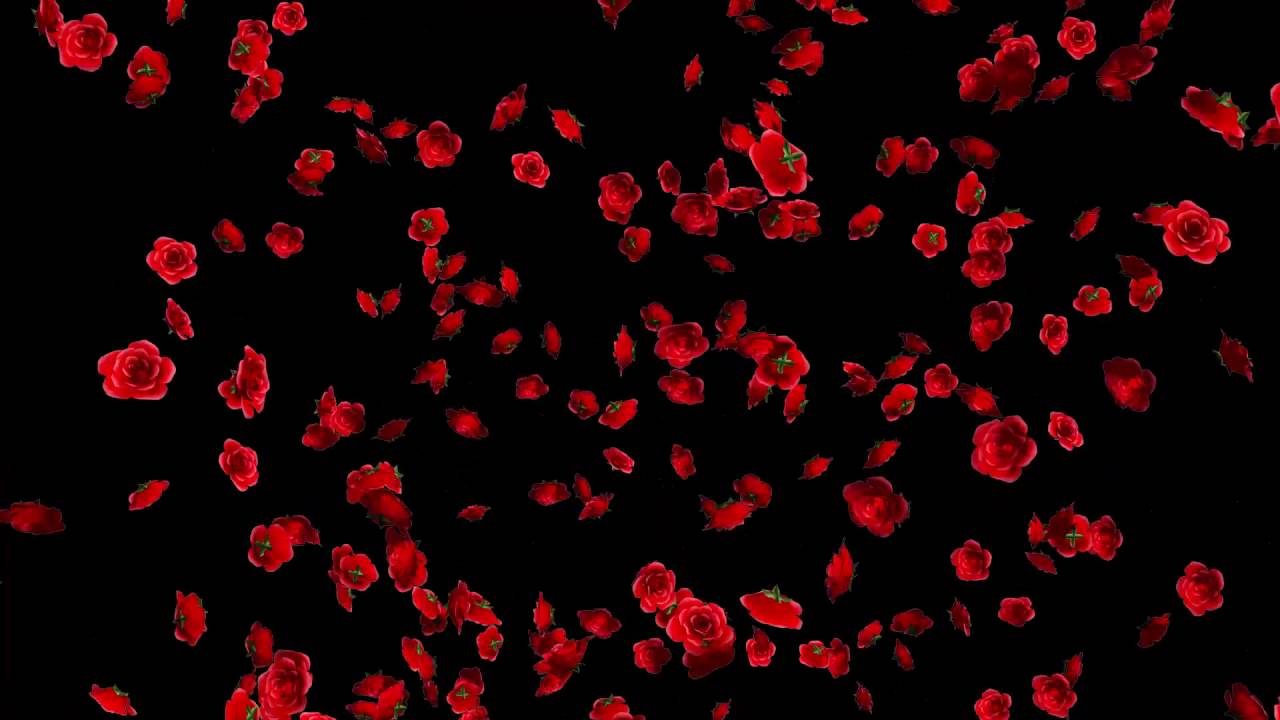The image features a dramatic display of hundreds of vibrant red roses set against a completely black background. The roses appear to be suspended in midair, as if floating or falling into a dark void. Each flower is richly detailed with multiple petals, and though most are stemless, some display green, cross-shaped leafy stems. These green elements punctuate the sea of red, adding texture and contrast to the composition. The roses vary in size and orientation, creating a random, natural arrangement that enhances the sense of depth and movement in the image. Overall, the picture evokes a feeling of surreal beauty, with the cascading roses standing out strikingly against the black backdrop.